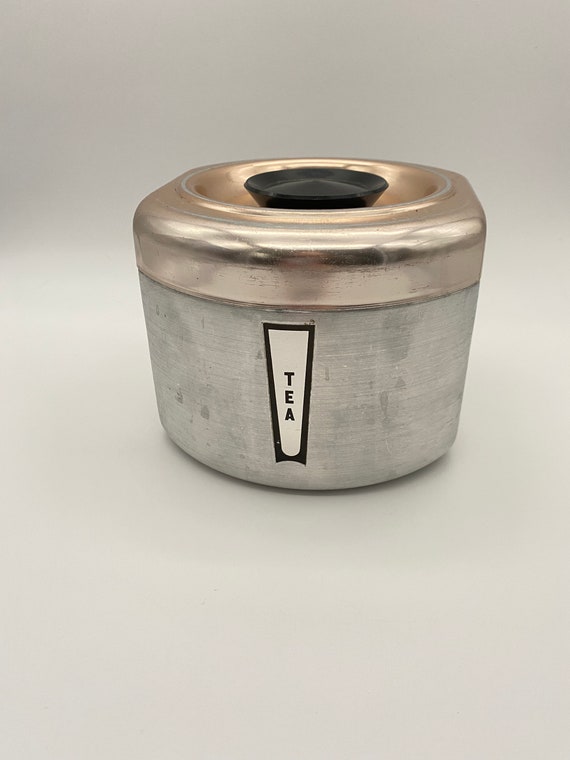The image depicts a simple, cylindrical, stainless steel teapot with an antique appearance, set against a neutral white-gray background. The base of the teapot is silver in color, evoking a potentially frosted or cold look, which is accentuated by the sleek, shiny finish. A vertical, white label edged in black and marked with the word "TEA" in bold black letters adorns the side of the teapot. The lid, contrastingly copper-toned, features a prominent, round black handle atop, emphasizing its utility and rustic charm. The subdued background serves to highlight the reflective quality of the stainless steel body and the striking details of the copper lid, making these elements stand out prominently.